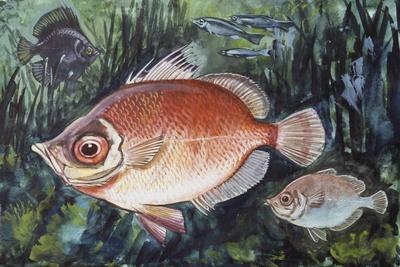The image depicts a richly detailed underwater scene, featuring multiple fish against a backdrop designed to evoke the appearance of seaweed and an under-the-sea setting. Central to the painting is a large brown and white fish with a scaly texture, several fins, and a prominent dark eye, shown in a side profile facing left. This fish, resembling a trout or sockeye salmon with a rounded body and smaller tail, is painted in a golden-brown hue with a whiter belly. Just below this central fish is a much smaller, similarly textured and finned grayish-brown fish. Above these two central fish are three sleek, silvery grayish-black fish that appear to be sardines or minnows, forming a small school. In the upper left-hand corner of the painting, there is an elegant, black angelfish with flowing fins. The background features a mix of greens, blues, grays, and blacks, skillfully painted to resemble seaweed and seagrass, enhancing the natural underwater ambiance.